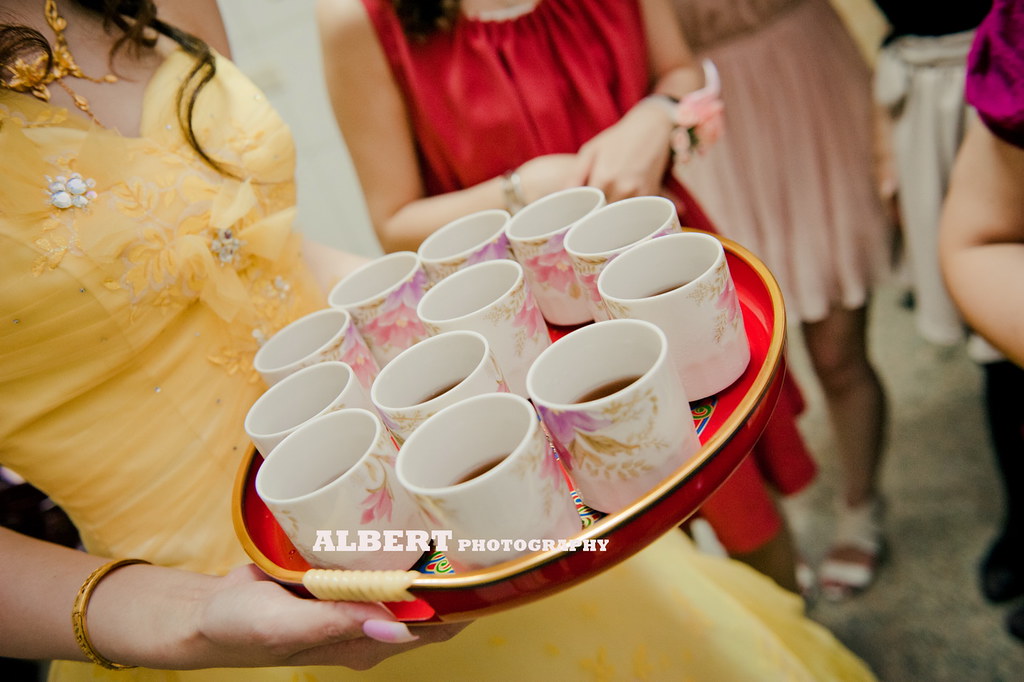This photograph captures a festive scene, possibly from a cocktail party or similar celebration. The central figure is a woman in a striking yellow dress, reminiscent of Belle from Beauty and the Beast, featuring a fitted bodice, perhaps adorned with jewels, and a slightly poofy skirt. Her accessories include a gold bracelet and a yellow necklace, and her medium-length, square-cut nails are painted pink. Strands of her dark hair hang gracefully down. She is holding a large, round red serving tray filled with twelve white mugs decorated with pink and green floral patterns; some of the mugs contain a brown liquid, likely tea or coffee.

In the blurred background, several other women in elegant party attire are visible. To the immediate right of the central figure stands a woman in a bright red dress with her arms held in front of her. Another woman, further back, is dressed in a pink mini dress paired with white strappy shoes. Also partially visible is a woman in a black top, white skirt, black leggings, and black shoes. The photograph has a professional touch with the inscription "Albert Photography" in white text at the bottom center. This detailed and vibrant capture presents a lively gathering of well-dressed women at what appears to be a joyous social event.